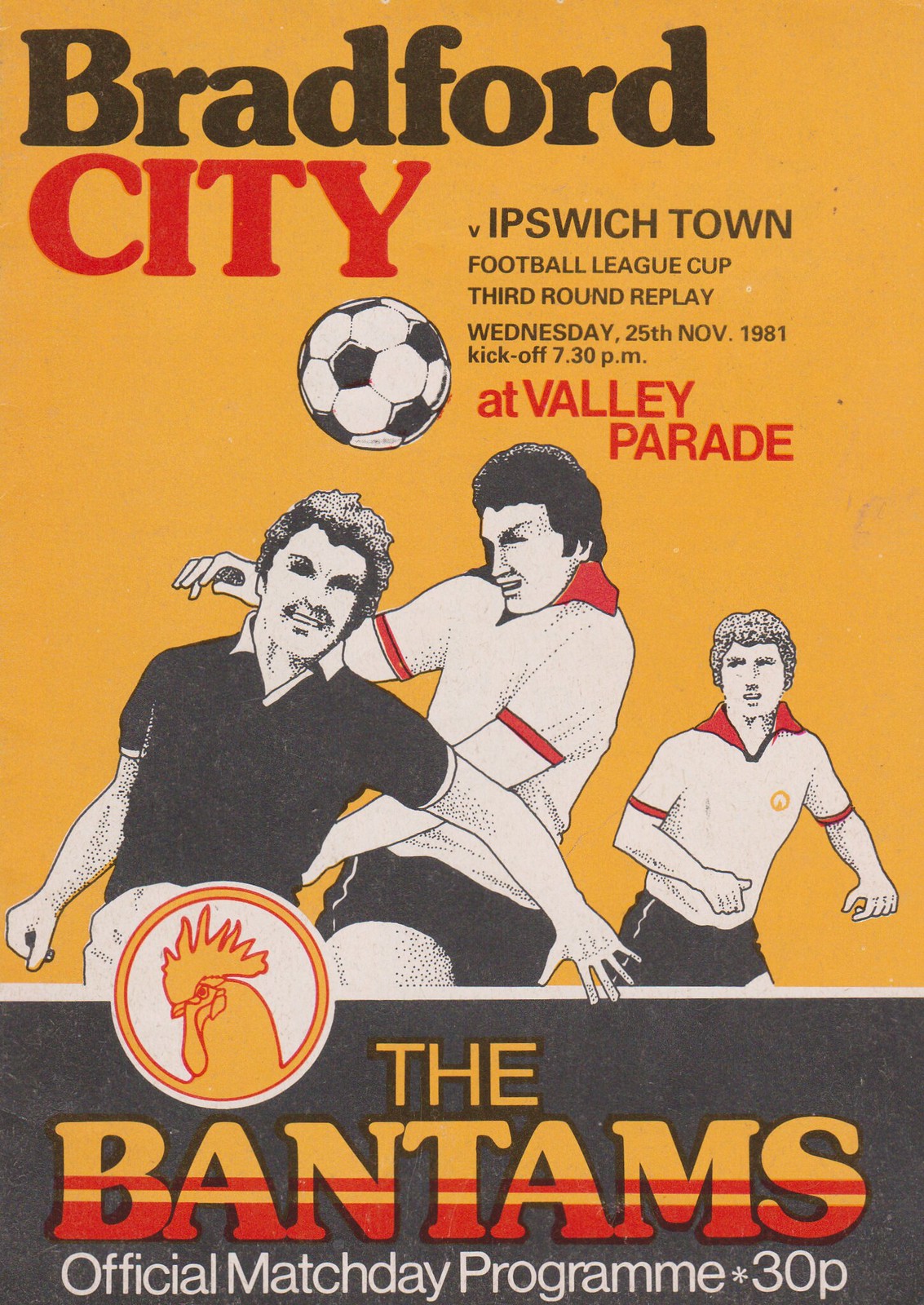This image features an official match day program from a soccer match. The program has an orange cover with the header stating, "Bradford City vs Ipswich Town, Football League Cup, Third Round Replay, Wednesday, 25th November 1981, Kickoff 7:30 PM at Valley Parade." In the center of the cover, there is an illustration of three soccer players actively engaging with a soccer ball that is suspended in mid-air. Two of the players, dressed in white shirts with red collars, appear to be attempting a header, while a third player, outfitted in a black shirt with a white collar, watches in the background. Near the bottom of the program, there is an emblem featuring an orange rooster inside a circle. Below this emblem, in orange and red ombre font, it reads "The Bantams." The footer also specifies that this is the "Official Match Day Program" sold for "30P." The background of the program is noted to be yellow, creating a striking contrast with the illustrations and text. 

This detailed composition underscores the historic and spirited atmosphere surrounding the Bradford City football match of 1981.